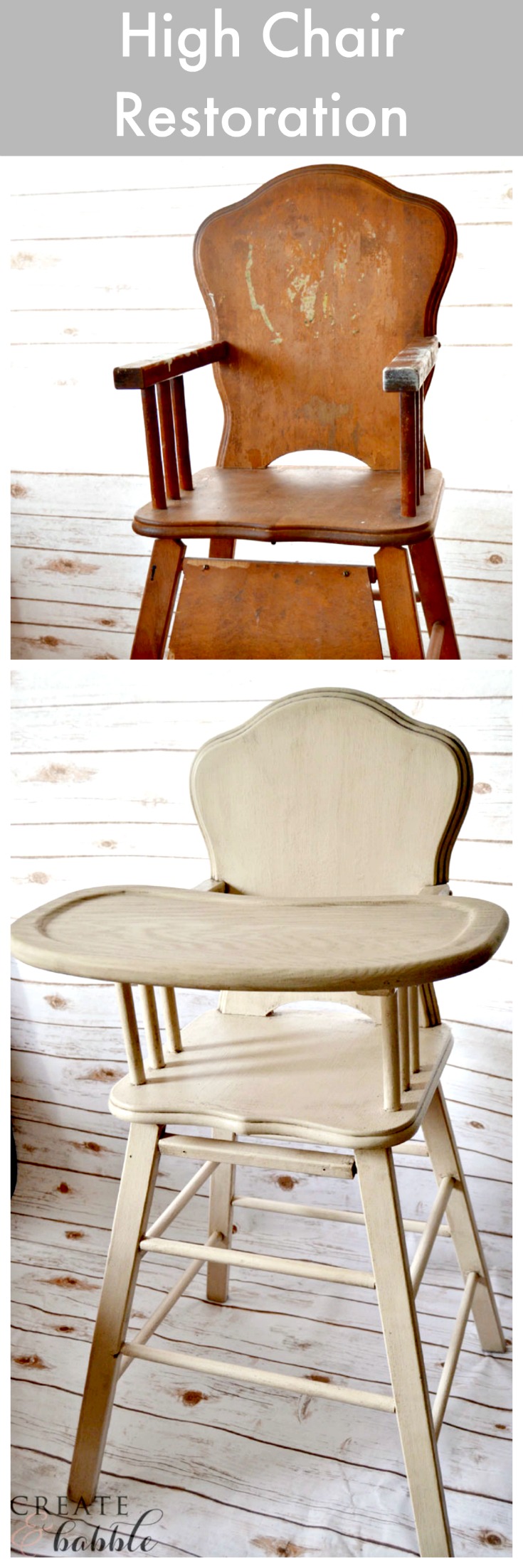The image features two distinct highchairs, positioned one above the other, on a white wooden floor with visible knots, set against a matching white wood panel background. The upper section showcases a highchair crafted from dark wood with evident white marks on its back, and it lacks a tray but includes armrests. Above this chair, "Highchair Restoration" is inscribed in white font on a gray background. In contrast, the lower section displays a restored highchair of lighter wood with a built-in tray and white legs. Both highchairs cast shadows against the background, suggesting natural, well-lit conditions. The word "Create in Babel," with "Babel" in cursive, appears in the lower left corner, signifying an artistic or restoration project.